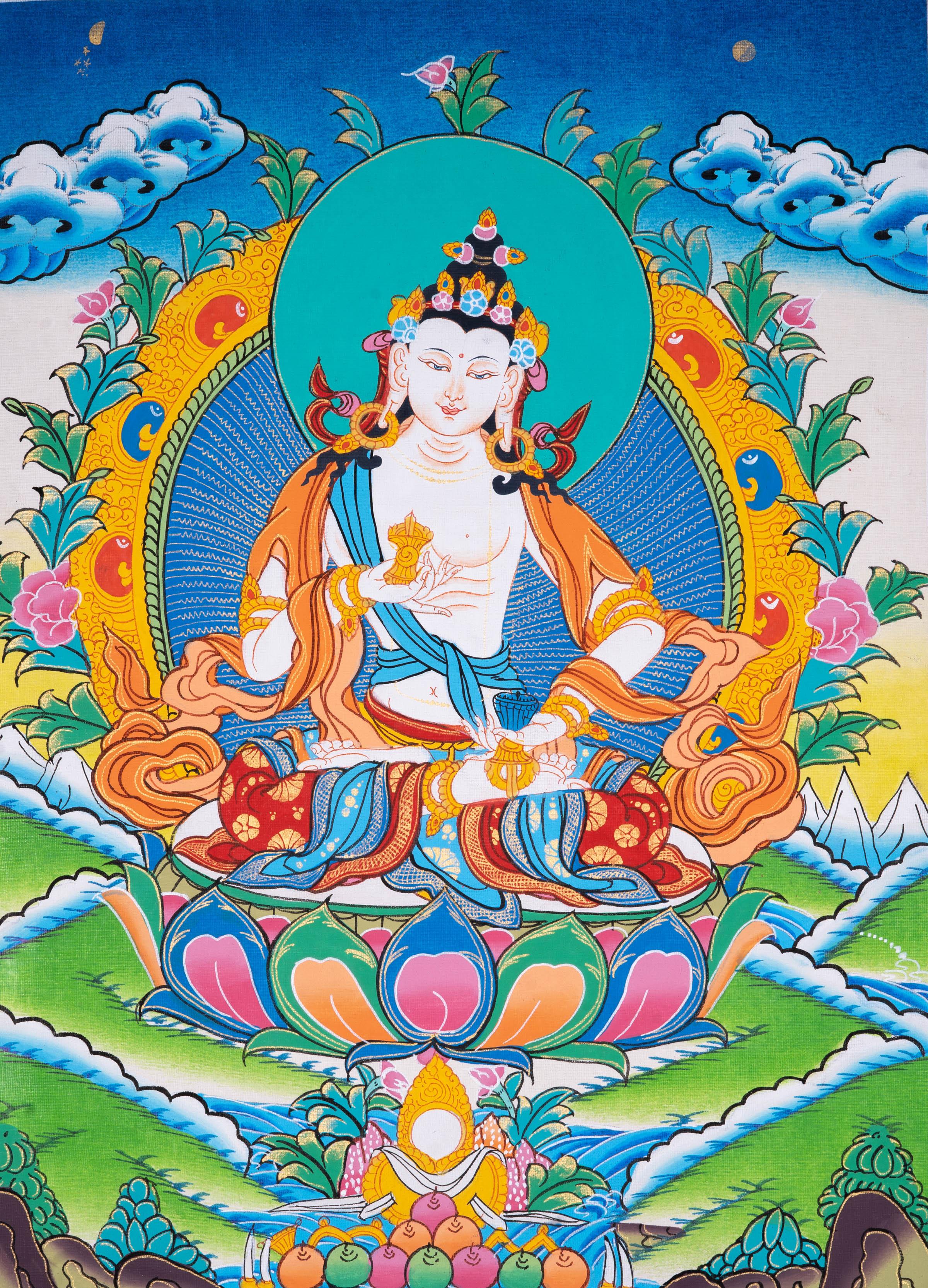The image is a vibrant and detailed portrait of Vajrasattva, the primordial Buddha, rendered in a highly colorful and almost psychedelic style. The figure is depicted with a bare, pink-toned torso, wearing an ornate ensemble that includes a flowing, stringy robe with a blue sash, red and blue scarves adorned with gold medallions, and a yellow cloak draped around the shoulders. Vajrasattva sits in a meditative posture with legs crossed, atop a large, round cushion made of alternating lotus flower petals in hues of blue, pink, green, and yellow, highlighting a white base.

His head is adorned with a headdress featuring dark, triangular, floral, and jewel-encrusted elements, including a gold crown studded with blue and green gems, and a bindi on the forehead. Gold earrings stretch his lobes, adding to his regal appearance. Behind his serene, smiling face is an elaborate halo effect comprising dual concentric circles: an inner aqua circle and an outer gold circle with intricate leaf ornamentation and blue ridges.

The setting is outdoors, indicated by the sky and clouds in the background, with green elements in the foreground likely symbolizing grass. Scattered multicolored shapes and fruits enrich the composition. Vajrasattva holds a gold item close to his chest, further emphasizing his divine status. This hand-drawn and meticulously painted piece merges elements of cartoonish art with exotic Indian Buddhist motifs, creating a richly detailed and spiritually evocative image.